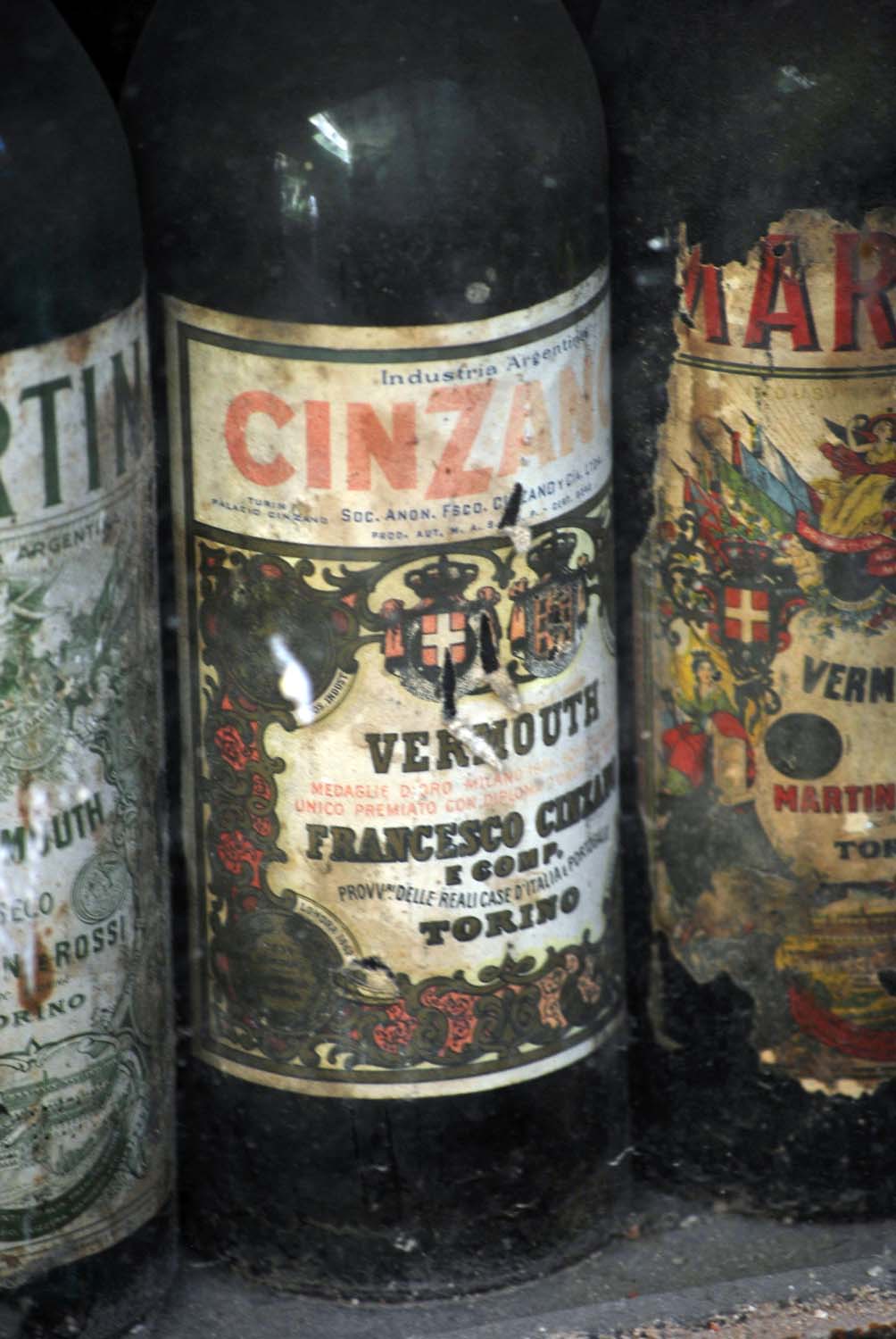This detailed caption describes an image that features three very old, almost black glass bottles prominently displayed. The bottles are labeled as vermouth but their labels are worn, stained, and peeling, adding to their aged appearance. The black and red labels on the left and right bottles are partially visible due to the framing of the photo, but it's evident that one says "Martin" and the other shows "RTIN," likely indicating "Martini."

The center bottle’s label, though faded, is more readable. It is primarily white with a black border and contains various stylized images, including a red shield with a white cross topped by a black crown. In red letters at the top, the name "Cinzano" (slightly cut off) is evident. The text on the label includes "Industria Argentina," "Vermouth," and "Francesco Cinzano," followed by "Torino." The design features intricate floral patterns in black and red, which border the entire label. This intricate detailing and the visible text help identify the bottle as a product of Cinzano, a known vermouth producer.